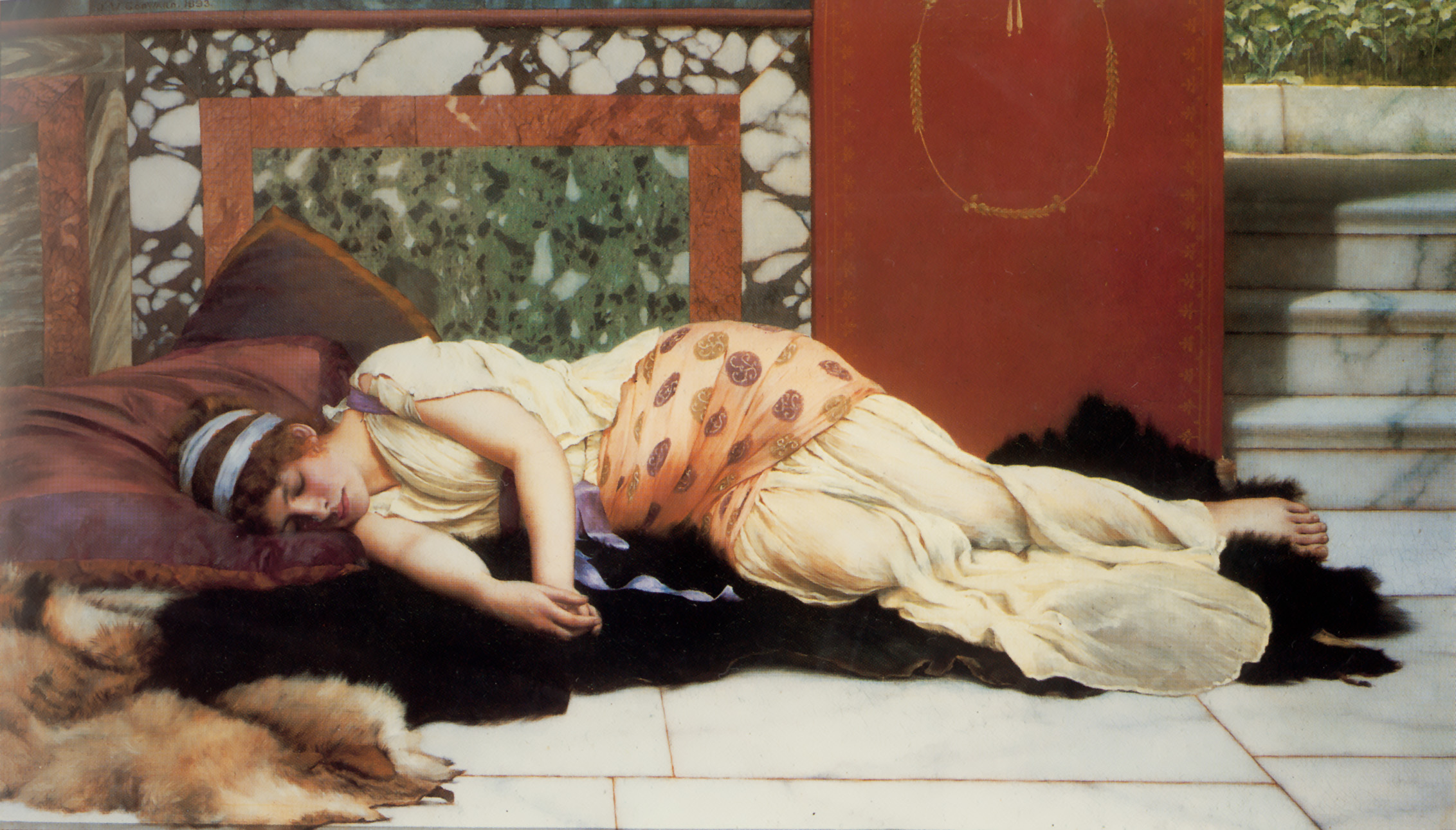The image depicts a young woman lying on a rectangular, horizontally aligned marble floor, resting on her right side with her head positioned on the left and her feet on the right. She appears to be sleeping, with her eyes and mouth closed, and her short curly brown hair partially covered by two bands of fabric that resemble a knitted cap. Her arms extend out in front of her, and she is barefoot. She is dressed in a full-length white gown reminiscent of a nightgown or dress, adorned with an orange-patterned wrap around her waist that features large brown polka dots.

Her head rests on decorative pillows, and she lies atop a bear skin rug, which is black and brown, with another animal skin, possibly a fox, beside her. The floor beneath them is made up of white square tiles. In the background to the right, there are three marble steps with a marbled pattern in white and gray leading upwards. Beyond the steps, a red decorative railing with green accents and an open door is visible, through which the upper right corner reveals a glimpse of trees, suggesting an outdoor garden area. The overall scene is rich in textures and details, offering a sense of serene repose in a luxurious setting.